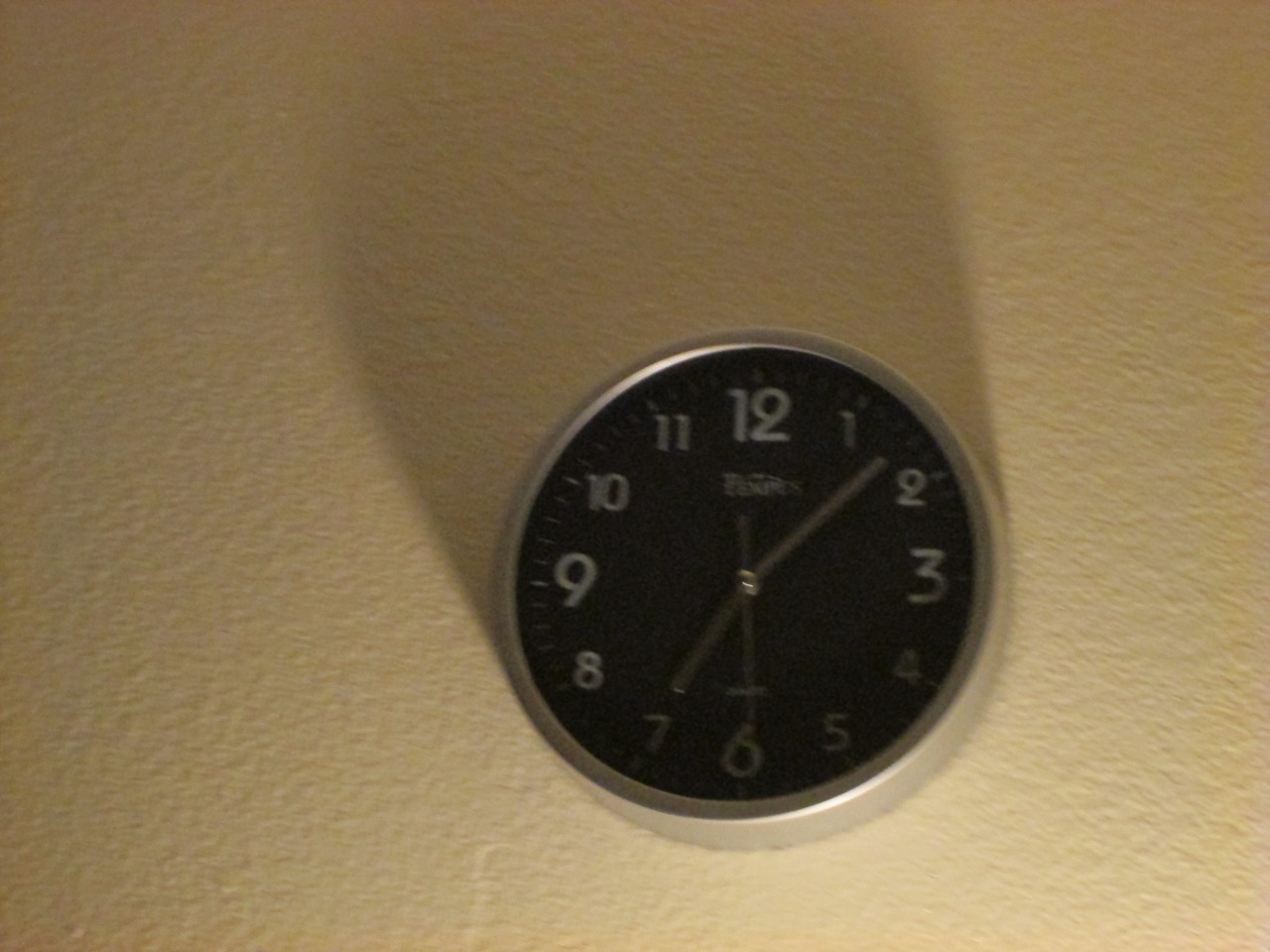This is a photograph of an old-style analog clock hanging on a textured beige wall, reminiscent of a 70s house interior. The clock features a silver metal frame encircling a black face with silver numbers. The 12, 3, 6, and 9 are notably larger than the rest of the numbers. The clock indicates a time of approximately 7:08 and 30 seconds, though it's unclear whether it's AM or PM. The hour and minute hands appear to be made of metal, with some descriptions suggesting the presence of red hands. The image is somewhat dark and grainy, suggesting poor quality, with a noticeable shadow extending up and to the left of the clock, cast by a light source positioned below, likely a desk lamp. An additional light glare on the bottom right of the metal frame confirms this lighting setup. The clock is slightly off-center towards the left in the composition of the photograph.